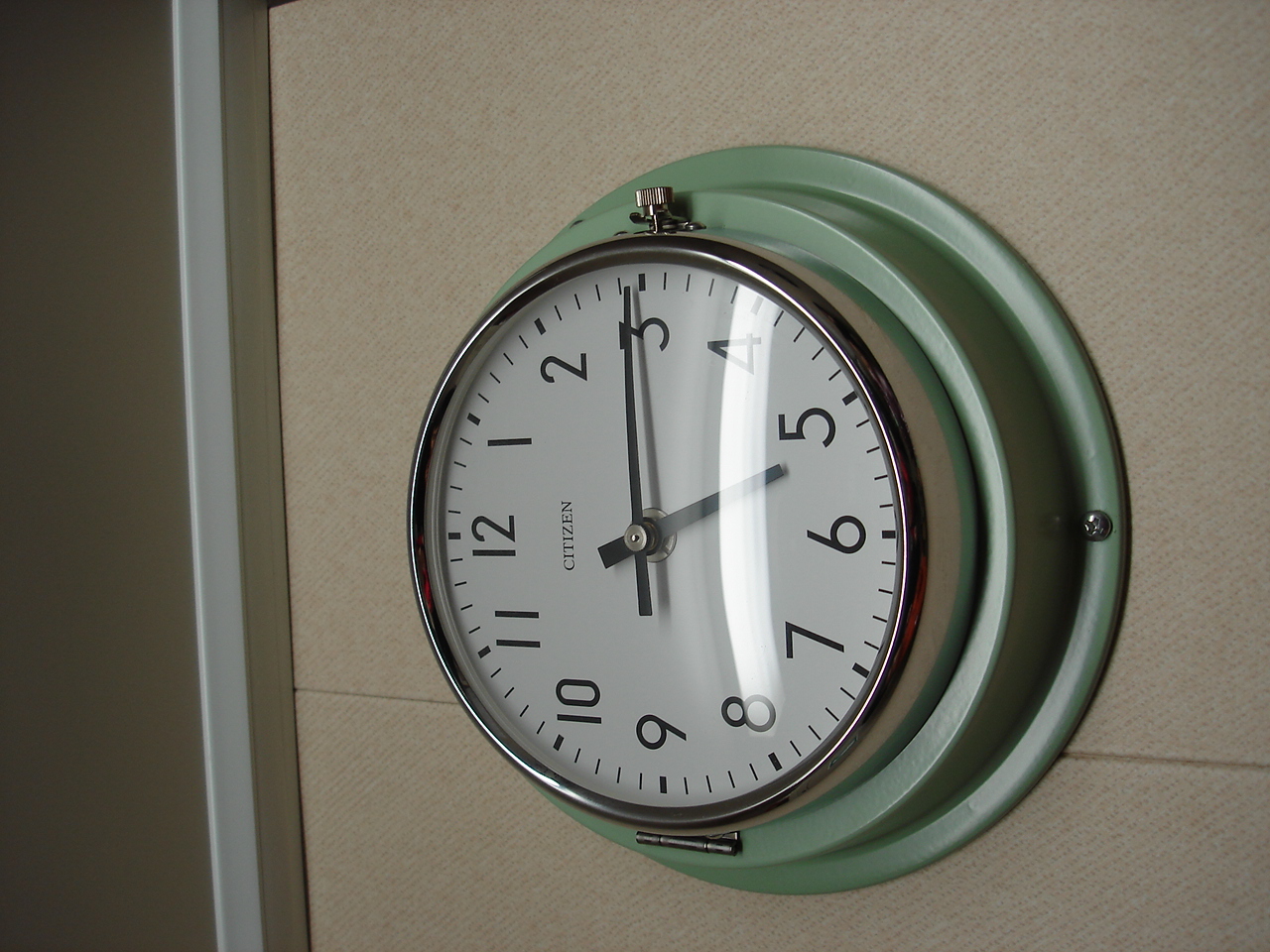A detailed and cleaned-up caption could be:

"An image depicting a clock with a mint green casing, mounted on a textured tan wall. The wall is segmented, indicated by a prominent line running through it. The photograph is rotated 45 degrees, causing the clock to appear tilted with the '9' at the bottom. The clock displays standard English numerals, and the time reads nearly 5:15."